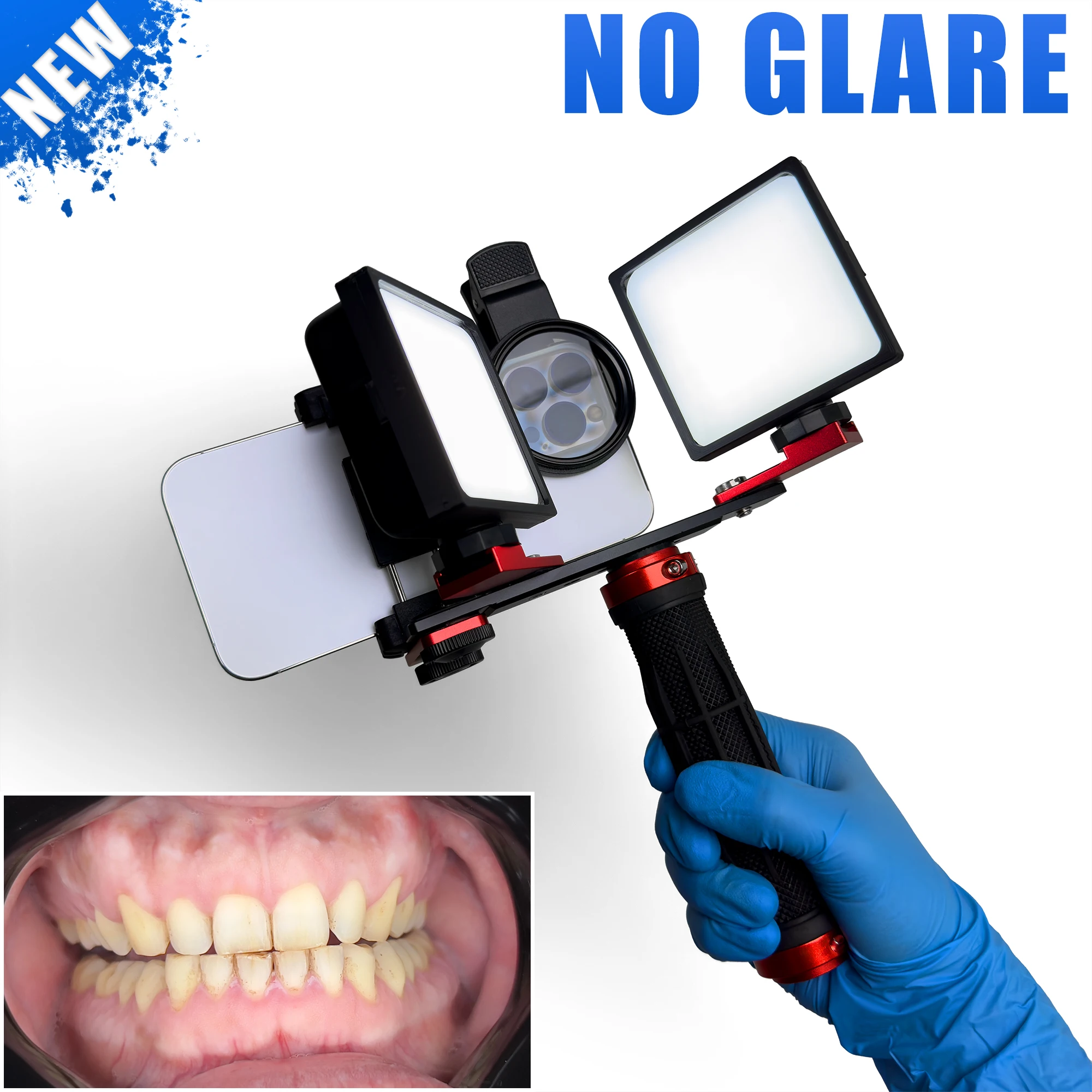This image is an advertisement featuring a specialized dental photography tool designed for capturing high-quality images of patients' teeth. Set against a white background, the product resembles a short selfie stick with a red and black handle and multiple mounts at the top. Two of these mounts hold lights positioned perfectly to illuminate the oral cavity, while a central mount connects to a cell phone, equipped with a lens and clip, to ensure optimal imaging without glare. In the upper left corner, the word "NEW" appears in bold white letters against a bright blue splash, and "NO GLARE" is prominently displayed in blue text in the upper right corner. A blue latex-gloved hand is holding the device, demonstrating its usage. In the lower left, an example photograph showcases a detailed view of someone’s teeth and gums, illustrating the tool's effectiveness in dental photography.